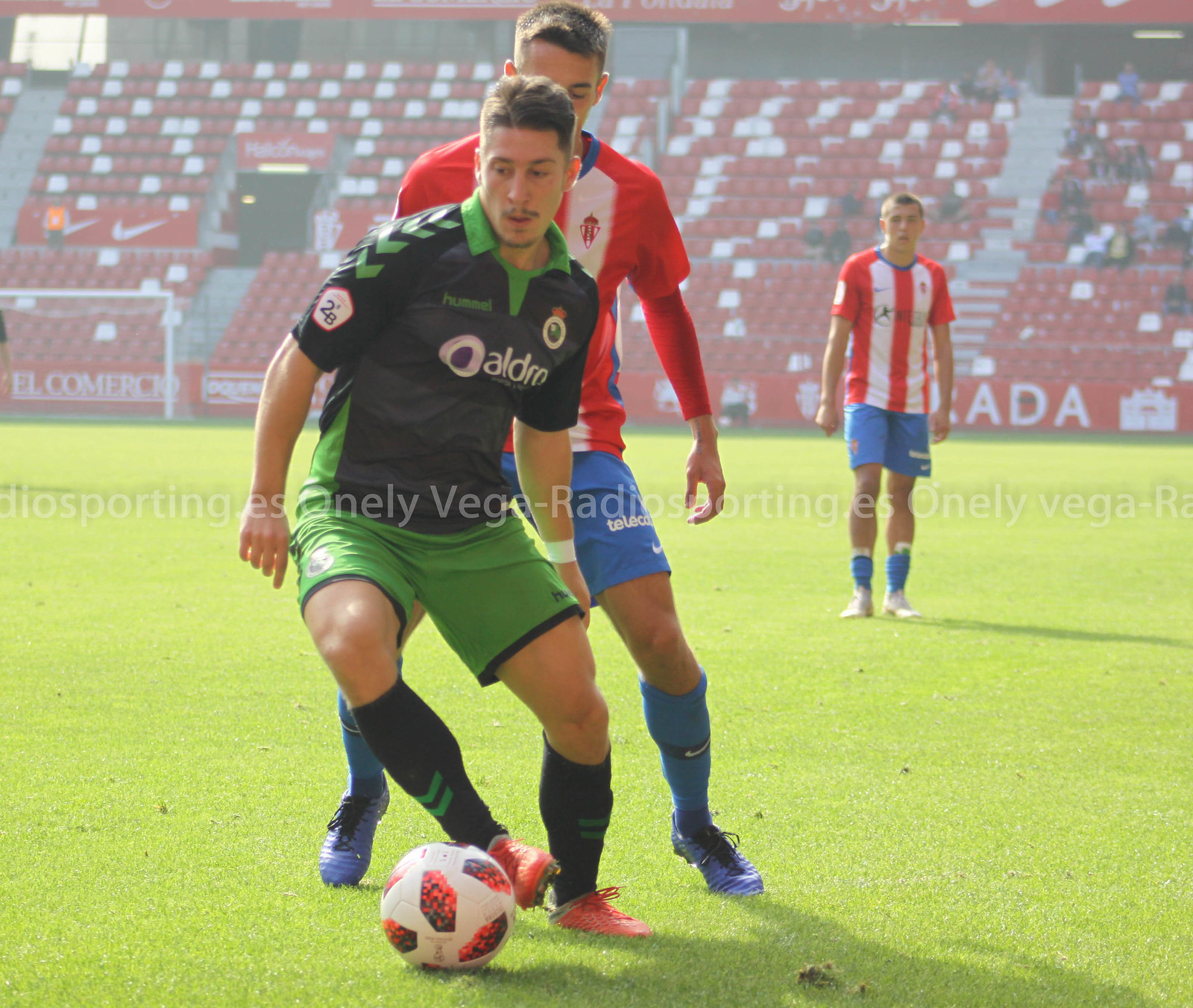In the foreground of the image is a competitive soccer match taking place on a vibrant green field. Central to the action is a player in a black and green jersey, dribbling the soccer ball with precision. His uniform includes green shorts, black socks, and red cleats, and the shirt has "Aldro" emblazoned on it. Directly behind him, an opposing team member clad in a red and white vertically striped jersey with blue shorts, blue socks, and blue cleats is in pursuit, attempting to intercept the ball. Slightly further back to the right, another player from the same opposing team, wearing a matching striped jersey and blue shorts but with white cleats, is observing the play with an open-mouthed expression of concentration.

The background features the empty white soccer net positioned just to the far left of center. Above the field, the partially filled stadium seating is visible, characterized by its red seats and the presence of a few spectators, suggesting perhaps a practice session or a match with a low turnout. The stands form the upper half of the image, framing the dynamic scene below. The image also includes a watermark with the text "Dio Sporting OnliVega, Radio Sporting OnliVega", indicating the company that captured this lively moment of athletic competition. The bright sunlight casting shadows of the players emphasizes the clear, sunny conditions of the day.